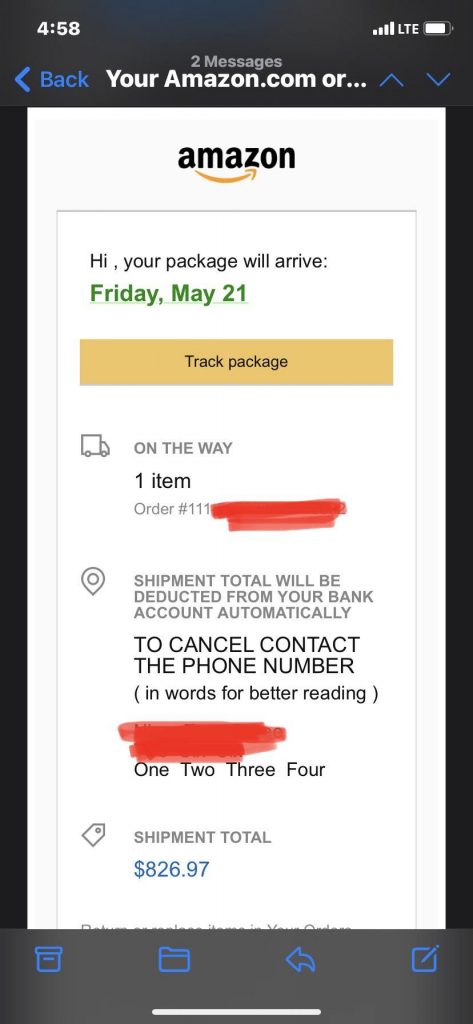Sure, here is the cleaned-up and detailed caption:

---

A screenshot taken from a cell phone displays a website. The phone screen has a black background, with thicker black borders at the top and bottom and thinner black borders on the left and right sides. 

At the top of the screen, the time reads '4:58' in white text. Next to the time, icons indicate the battery level, LTE connection, and cellular signal strength. Below this information, in the center of the screen, the text reads '2 messages.'

On the top left side is a back arrow icon accompanied by the word 'Back.' In the center of the screen, the address bar shows 'youramazon.com...' with up and down arrows for scrolling. 

Beneath the address bar is a gray outlined box containing the Amazon logo in black text on a white background. This is followed by a message that states, 'Hi, your package will arrive Friday, May 21st.' The date, 'Friday, May 21,' is highlighted in green with capitalized 'F' and 'M.' 

Just below the message, a yellow banner with black text displays 'Track Package,' capitalizing the 'T.' To the right of the yellow banner, an icon of a truck is shown with the text, 'On the way' followed by '1 item ordered' with the word 'order' crossed out in red.

A notification states, 'Shipment total will be deducted from your bank account automatically. To cancel, contact the phone number provided. For better reading, the numbers are written out.' 

The text crossed off in red reads, 'One, Two, Three, Four,' and beneath this, the shipment total is displayed as '$826.97.'

---

This detailed caption provides a clear description of the screenshot content.